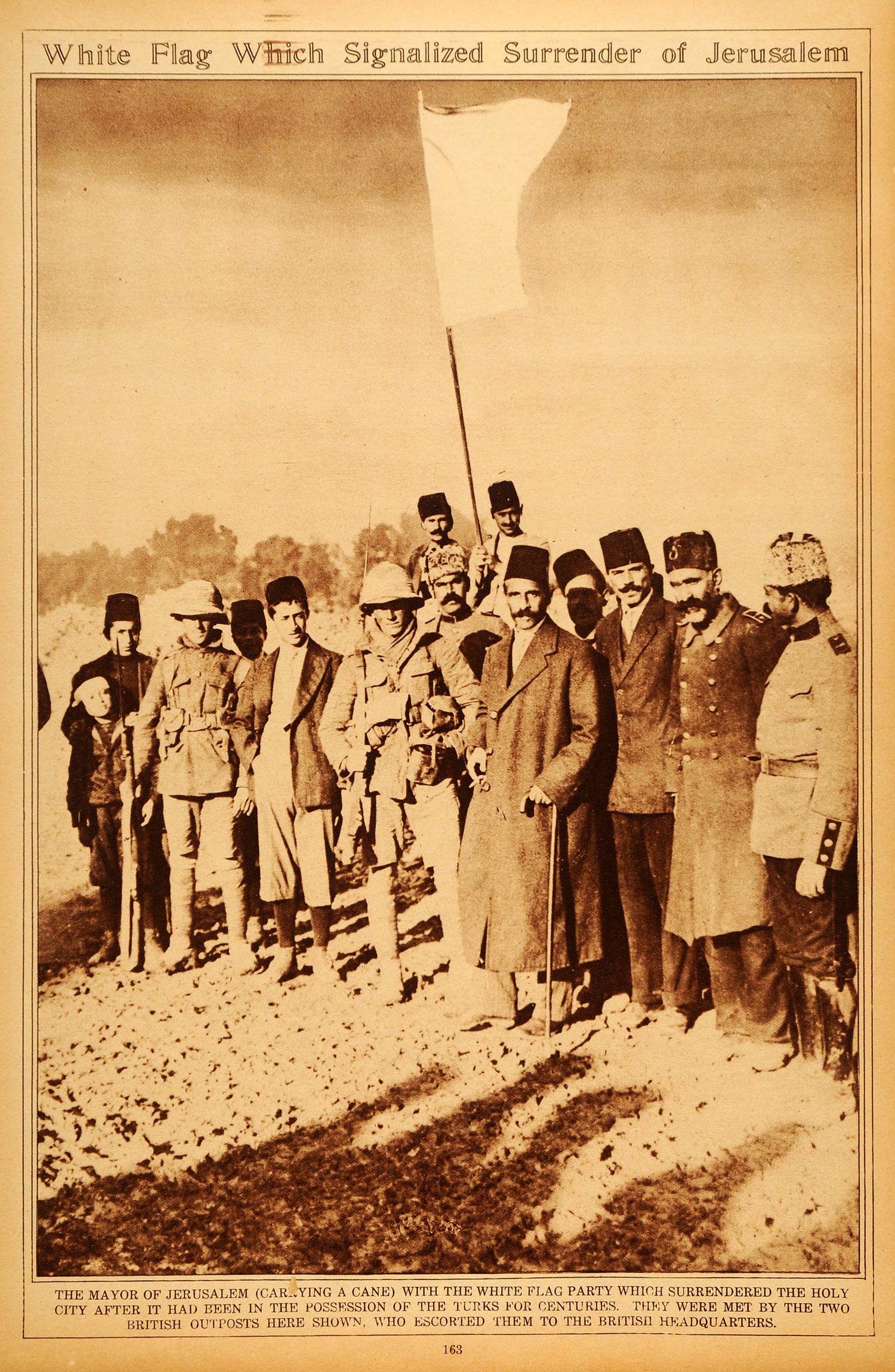This sepia-toned photograph is an aged image, likely from a newspaper or book, depicting a historic moment in Jerusalem. The text at the top reads, "White flag which signaled surrender of Jerusalem." The scene showcases a mix of British soldiers and Turkish men. The two British soldiers are identifiable by their old-style uniforms, complete with heavy canvas jackets adorned with numerous pockets, belts with pouches, leggings, boots, and helmets. They are holding rifles. The Turkish men, some wearing tall, rectangular hats like fezes and dark overcoats resembling navy pea coats with buttons down the front, stand alongside. There is also a notable figure in a lighter colored jacket and fez. The background shows one man holding a large flagpole with a white flag.

The gravelly, dirt-covered area on which they stand, further emphasizes the period setting of the event. At the bottom of the picture, the caption identifies the mayor of Jerusalem, holding a cane in his left hand, as part of the white flag party. This group surrendered the holy city after it had been under Turkish control for centuries. The text continues, "They were met by the two British outposts here shown, who escorted them to the British headquarters," affirming the British soldiers' role in the scene.